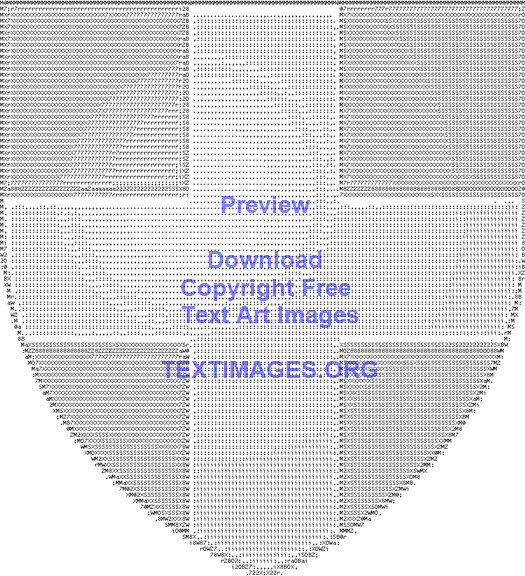The image features a shield with a flat top and curved sides that meet at a point at the bottom, forming a traditional shield shape. It is composed entirely of various ASCII characters, including asterisks, numbers like 7, question marks, and periods, arranged meticulously to generate a detailed graphic. The shield incorporates a prominent cross that spans the height and width of the design, with a denser border of characters framing it. 

The shield is rendered in black and white and stands out against a plain white background. Adding to the visual texture, the shield includes a circular highlight, giving it a dimensional appearance. Superimposed over this intricate text art are blue and purple words: at the top, it states "Preview", then "Download", and "copyright-free text art images." Below the shield, in uppercase purple letters, it reads "TEXTIMAGES.ORG." These texts serve as a watermark, possibly indicating the image as a sample or promotional material for a website offering text-based art.